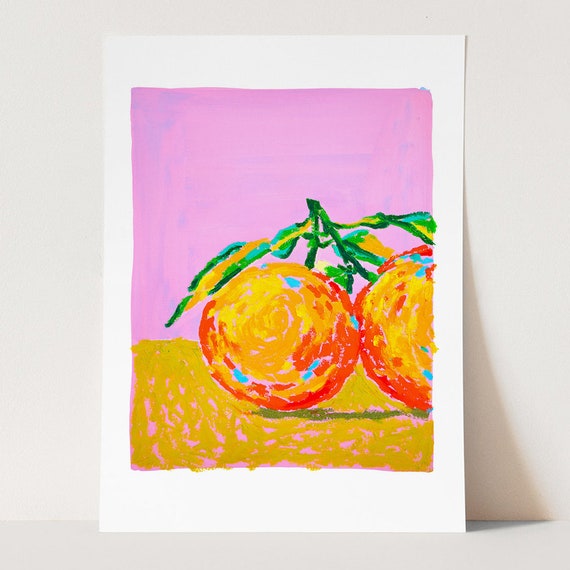This image showcases a vibrant painting propped against a white wall, casting a shadow to the right on both the wall and the ground. The artwork, rendered in a watercolor style, features a playful and colorful pop art or art deco theme on white paper. The upper two-thirds of the painting exhibit a vivid purplish-pink hue, reminiscent of a sky, transitioning into an orangish-yellow section at the bottom third. Dominating the center are two interconnected, round fruits—possibly oranges or tomatoes—characterized by their striking reddish-orange color interspersed with hints of blue and beige. Each fruit has a stem and leaves at the top, with one fruit partially cut off on the right side of the image, adding an element of intrigue to the composition.